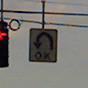In this very small, somewhat dim photograph, a complex scene is captured. Dominating the center is a white, square U-turn sign outlined in black with bold black lettering that indicates "OK" for making a U-turn. Adjacent to this sign, slightly to the left and partially cut off, is a traffic signal displaying a lit red left-turn arrow. This signal and the sign appear to be suspended from power lines that stretch across the image. The background sky has a subtle pink hue, suggesting the photo was taken at dusk. Details like the small curled wire beside the traffic light and the overall reduced visibility of elements due to low light add to the nuanced, detailed snapshot of a moment at a traffic intersection.